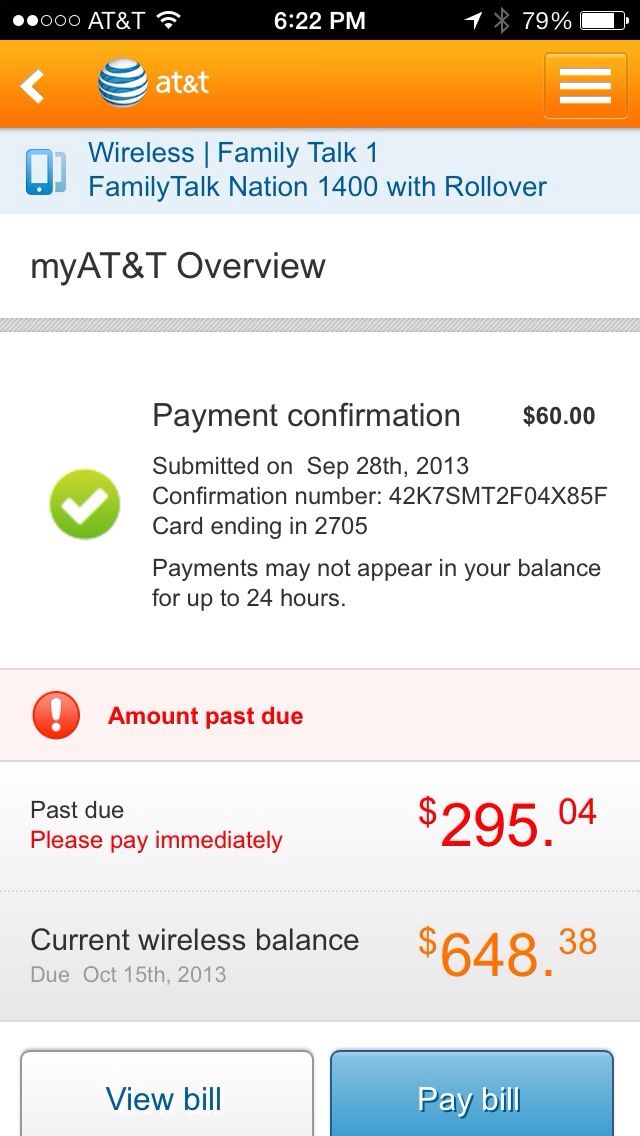This is a detailed screenshot of the billing page from AT&T viewed on a phone, showcasing various account and payment details. At the very top, the status bar shows the time as 6:22 PM, an internet connection icon, the Bluetooth symbol, and the battery at 79%. Below this, there is an orange bar featuring a white arrow pointing left, the AT&T logo, and a menu symbol. The following section has a light blue background with a blue cell phone icon and blue text that reads "Wireless Family Talk 1, Family Talk Nation 1400 with rollover."

The main section of the screenshot has a white background with black lettering stating "My AT&T Overview" separated by a gray bar. Below this, there is a payment confirmation with a green circle and a white checkmark, indicating a confirmed payment of $60 submitted on September 28, 2013. The confirmation details include a card ending in 2705 and a note that payments may take up to 24 hours to appear in the balance.

Further down, there is an off-white bar featuring a red circle with a white exclamation point and red text that reads "Amount Past Due." This section highlights an urgent past due amount of $295.04 in red, coupled with a warning to "Please Pay Immediately." Below this, a gray bar details the "Current Wireless Balance" with a due date of October 15, 2013, and an amount of $648.38 in orange. The bottom section includes two action buttons: a white one with blue text that says "View Bill" on the left, and a blue one with white text that says "Pay Bill" on the right.